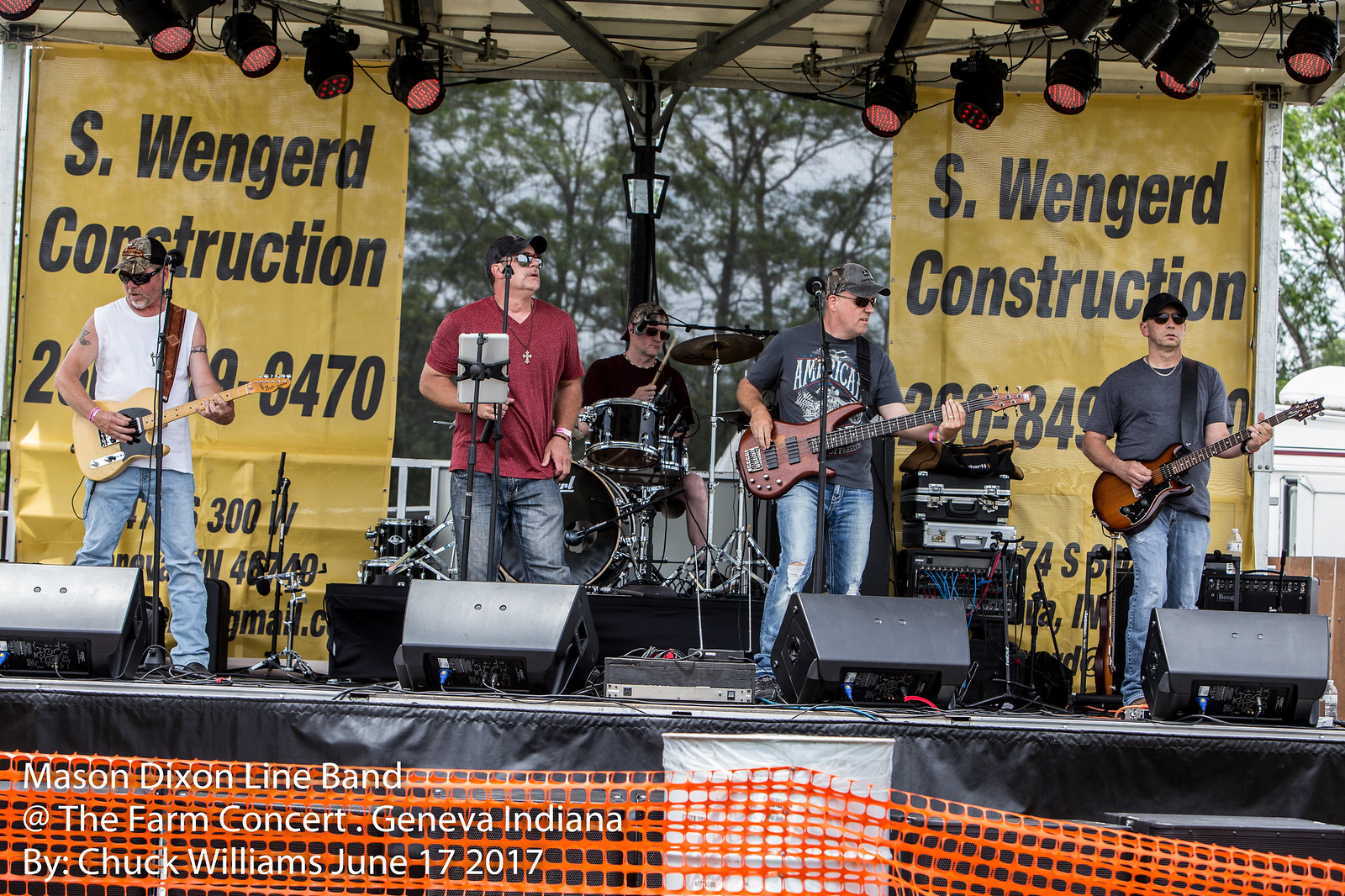This is a photograph capturing the Mason-Dixon Line Band performing live at the Farm Concert in Geneva, Indiana, on June 17, 2017. The image, taken by Chuck Williams, features five white male members aged between 40 and 50. All the band members are sporting baseball caps and sunglasses, contributing to their laid-back, country rock appearance. 

From left to right, the band members are as follows: the first is wearing a white tank top and playing an electric guitar. The next in line is donned in a red T-shirt and is the lead vocalist. The third member, in a black T-shirt, also holds a microphone and plays guitar. The fourth, clad in a black T-shirt, is the bassist. In the background, the drummer, dressed in a black T-shirt and shorts, anchors the rhythm section.

The stage is set with black flooring and is equipped with four speakers. Yellow or orange plastic fencing can be seen at the bottom, likely serving as a barrier for the audience. Two large banners are hung at the back, promoting S. Wengert Construction with a phone number, indicating sponsorship. The scene is framed by lush green trees, marking the event as taking place in spring or summer. Red lights shine down on the performers from above, highlighting the energetic ambiance of the concert. White text photoshopped onto the image provides details about the event and its date.